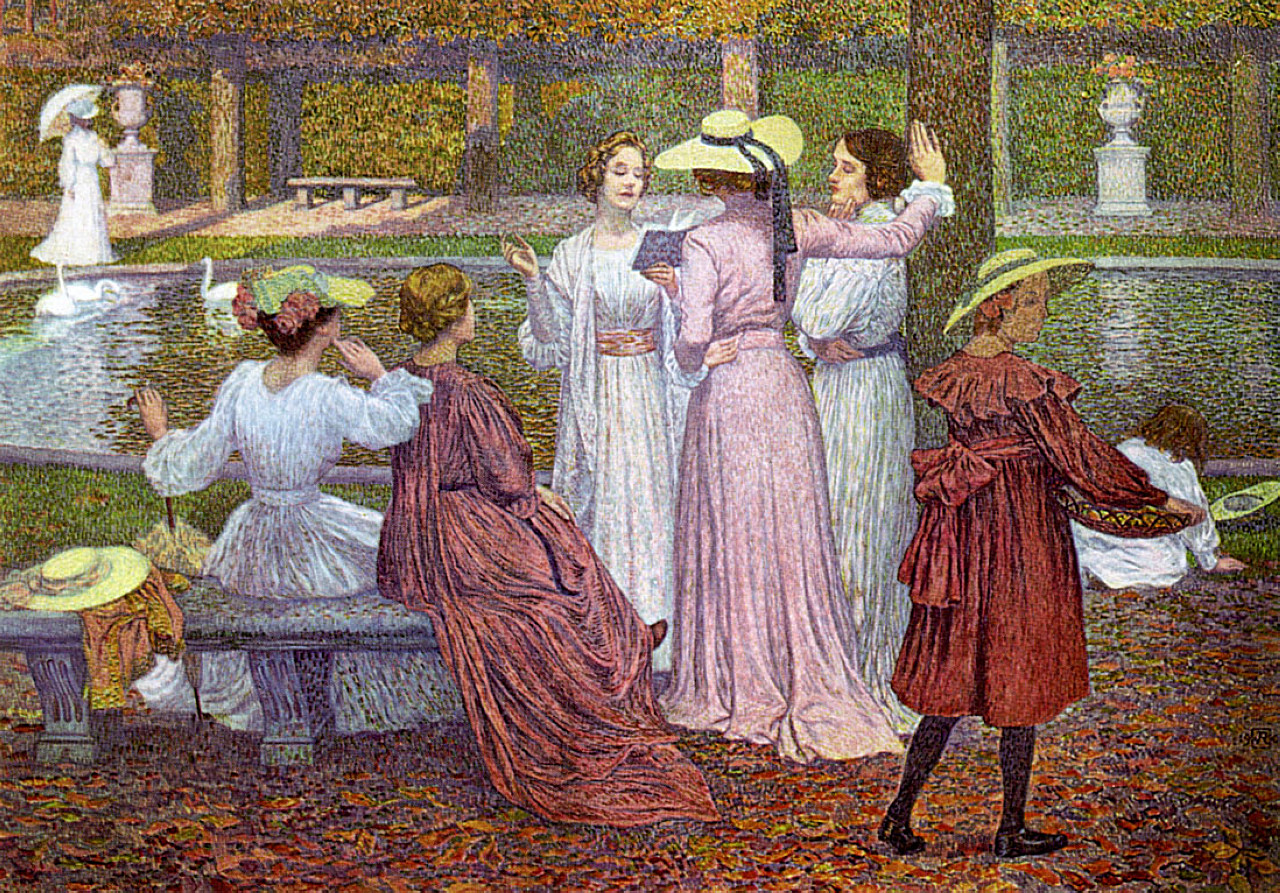The image depicts a highly detailed, impressionistic-style painting set in a lush garden, richly textured with pointillist dots. In the very center, three women form a focal trio. One, wearing a flowing pink gown and a wide-brimmed hat with a blue ribbon, stands with her arm resting on a tree trunk. Adjacent to her is another woman in a white dress with a pink sash, holding a book as if reading lyrics. The third woman, in a similar white dress, rests against the trunk. Their gestures and open mouths suggest they are singing.

To the left, on a stone bench covered in golden, red, and orange fallen leaves, sits a pair of women deeply engaged in the scene. One, wearing a white dress, sits beside a hay-colored bonnet, looking away. Next to her is a woman in a dark pink dress. Both observe the central trio with attentive expressions.

On the right, a smaller figure in a red dress with a broad-brimmed hat and black stockings heads towards the edge of the scene. Behind her, another young girl in white, with brown hair, kneels close to the ground, her gaze directed at the swans swimming in the nearby pond.

The serene background features lush green foliage, additional tree trunks, and elegant gray sculptures adorned with flowers. The landscape extends to a tranquil water body where white swans glide gently. The composition captures a moment of serene communion among this diverse group of women, set against a beautifully detailed, vibrant natural backdrop.